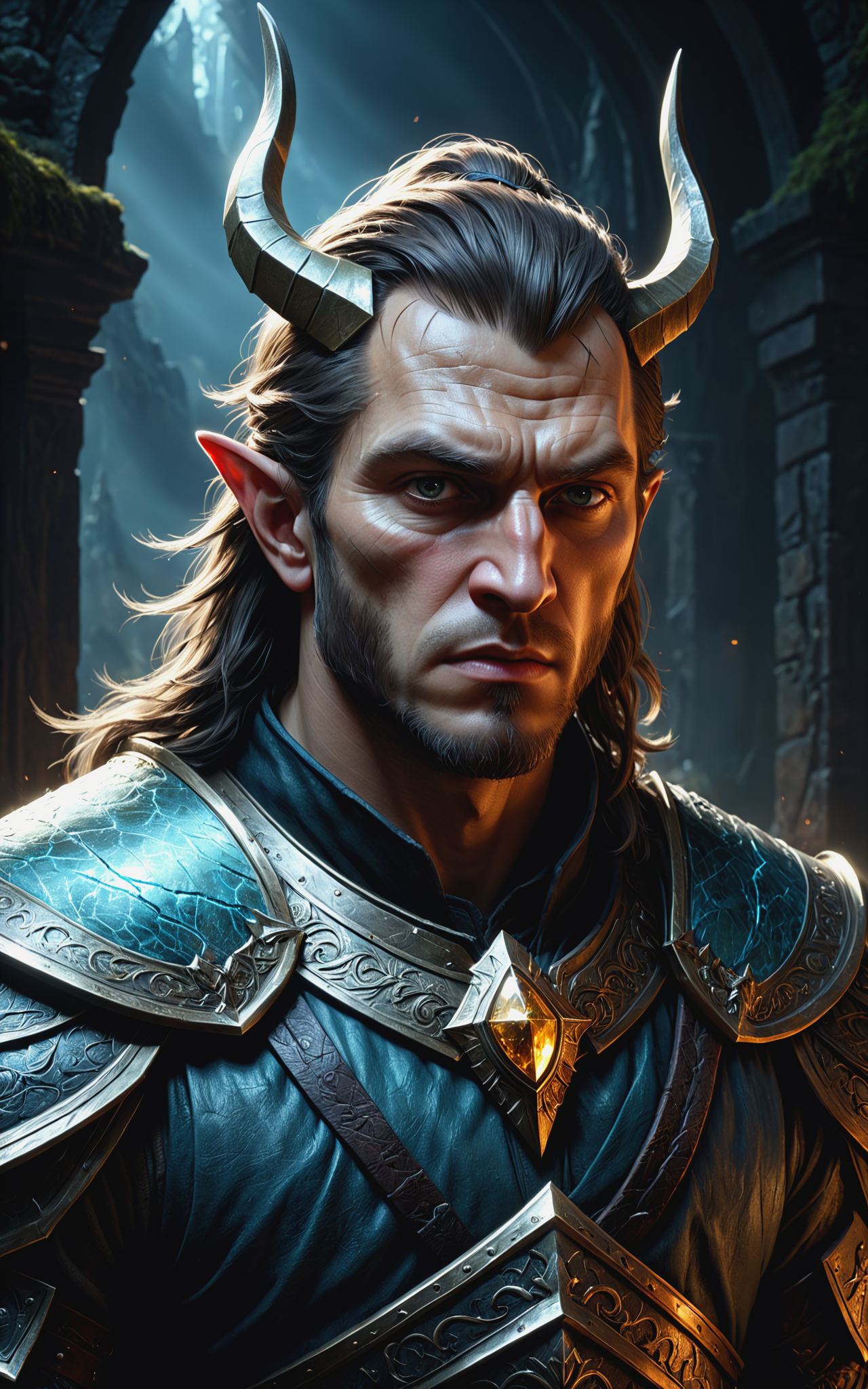This close-up, color image portrays a highly realistic, digitally rendered actor as a mythical character. He stands in front of a stone archway, backlit by sunlight streaming through a forest canopy. His long, brown hair and pointed elven ears frame his detailed face, featuring human-like, yet plasticky textures, including a wrinkled forehead, a beard, and a mustache. Large, gold horns protrude from his temples. He is adorned in elaborate armor consisting of a blue and silver armored jacket with metal shoulder plates, a chestplate featuring a diamond-shaped emblem, and metallic collar pins. His outfit also displays yellow leather elements, adding to his fantastical and heroic medieval appearance.